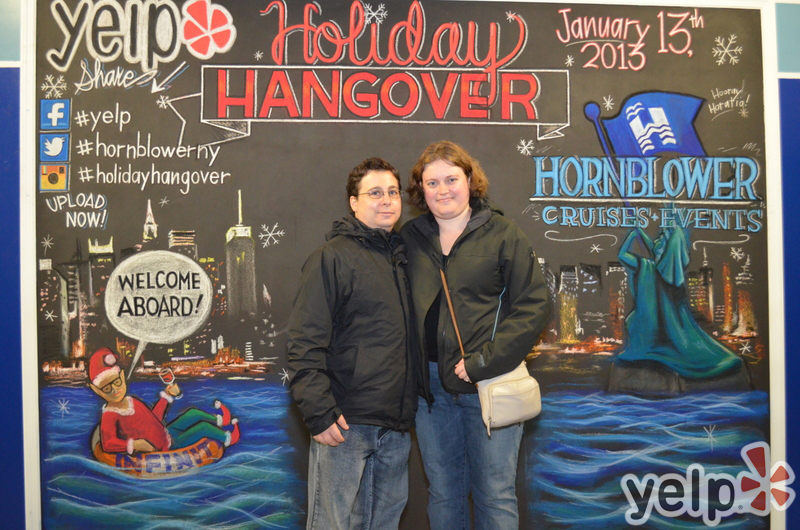Two brunette individuals donning black jackets and jeans stand in front of an elaborately designed backdrop that reads "Delft Holiday Hangover, January 13, 2013" and "Hornblower Creates a Difference." The man on the left side sports eyeglasses while the woman on the right holds a cream-colored handbag with a brown strap. Both are posed in front of a seemingly hand-drawn mural, which depicts the New York City skyline, complete with the Statue of Liberty holding a flag emblazoned with an "H." Snowflakes and floating bubbles are dispersed throughout the background, adding a whimsical touch. Below the cityscape, waves ripple through a body of water where a floating inner tube and a small lifeboat are illustrated; the lifeboat features a speech bubble stating, "Welcome Aboard." Hashtags such as #DelftHornblower.ny and #HornholidayHangover are visible, hinting at social media engagement. The Hornblower Cruises and Events logo is present on the right side, alongside additional text, including the Yelp logo and date.